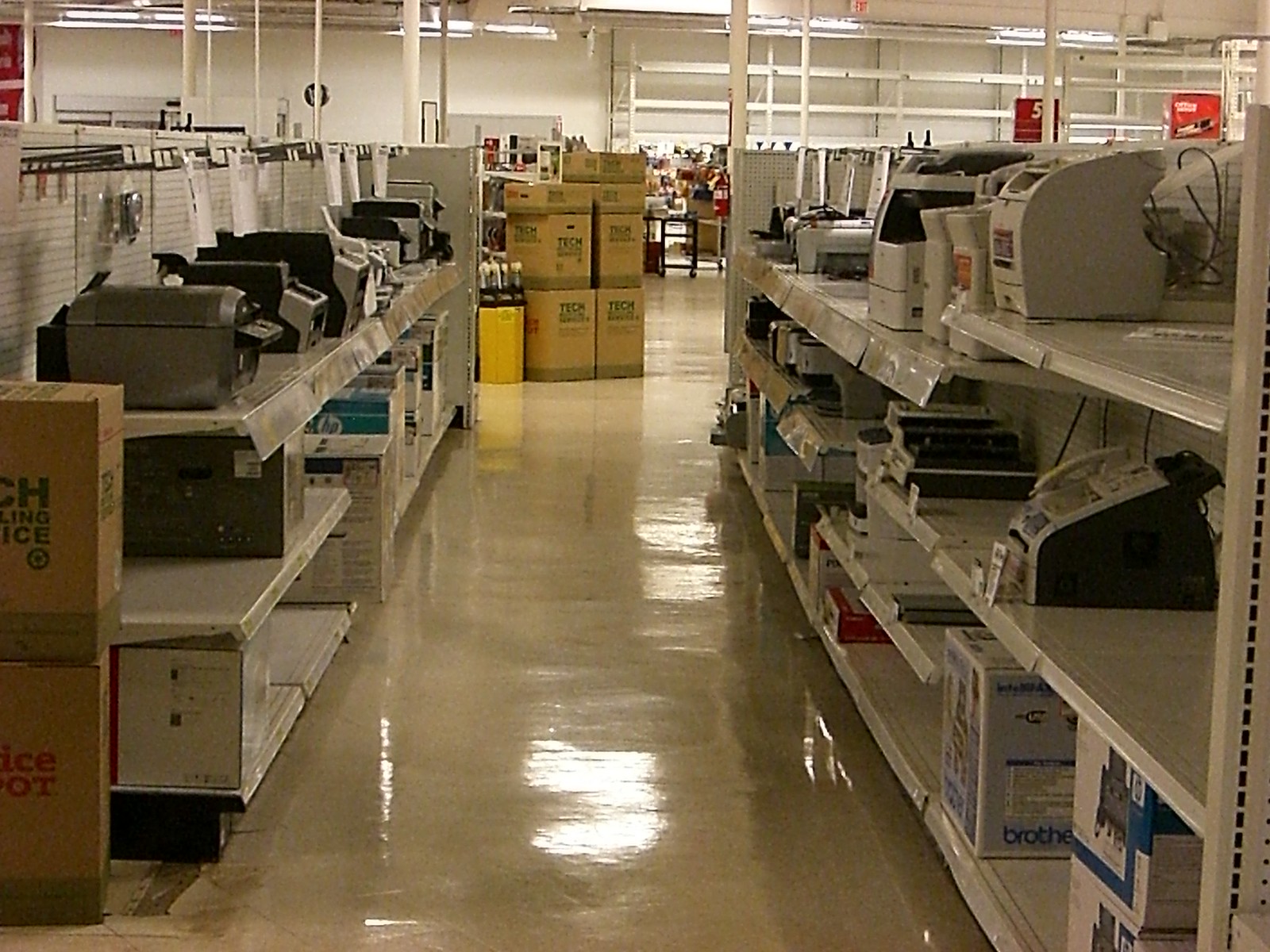The photograph captures the interior of a department store, reminiscent of an Office Max or Office Depot. Bright fluorescent lighting spans across the white ceiling, reflecting off the shiny, beige-tiled floor that appears recently polished. The aisle stretches forward, flanked by tan-colored, perforated shelving units on both sides. These shelves are lined with a variety of office equipment, primarily printers, copiers, and fax machines in white, black, and gray hues. The shelves are equipped with rod tags for pricing, with some prices visible.

To the left, two cardboard boxes, emblazoned with green text reading "TECH," are stacked. Similarly, on the right, there are more stacks of boxed items and office machinery. Further down the aisle, another stack of seven cardboard boxes is visible, reinforcing the store's focus on tech products.

White support poles interspersed throughout the store reach up to the ceiling, some adorned with red signage featuring images and text. One sign is partially legible, indicating a price starting with the number 5. Prominently, a white exit sign with red lettering hangs toward the center of the store, accompanied by additional fluorescent lights. The background reveals more shelves stocked with various products, encapsulating the orderly yet bustling atmosphere typical of a tech retail environment.